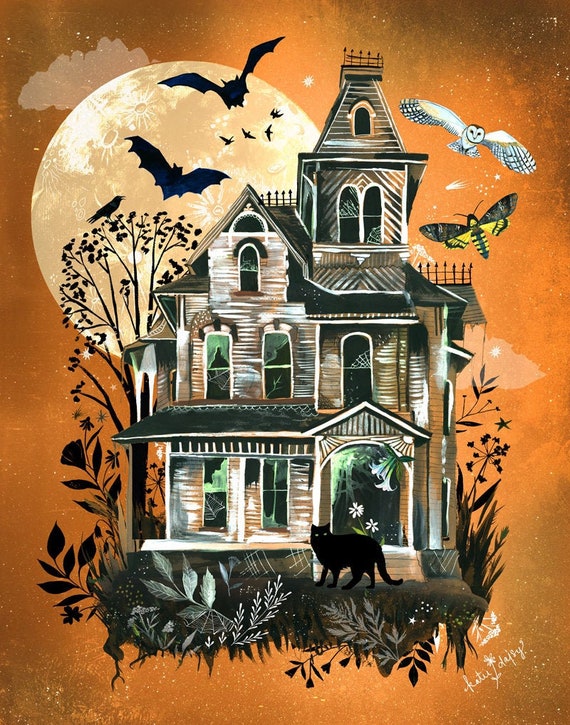This Halloween-themed image is a graphic design featuring a dark orange background and a massive, milky-colored moon dominating the upper left corner. Silhouettes of numerous bats are flying in front of the moon, adding to the eerie atmosphere. Below the bats, a Victorian-style, three-story haunted house stands as the central focus. The house is characterized by its various little windows, gables, and cobwebs in the broken windows and around the structure. A ghostly black cat with only its yellow eyes visible sits in front of the stairs leading up to the porch. Additionally, a white barn owl with its wings outstretched and a black and yellow moth hover above the house. Surrounding the house are neat floral and leaf arrangements, along with spiderwebs in the grass. A large tree with a crow perched on its branch adds to the spooky scene. The sky is filled with white starry dots and astral images, enhancing the haunting mood. An artist’s signature in white can be seen in the lower right corner, though it is not legible.